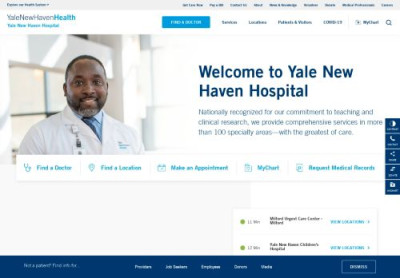Screenshot of a Yale New Haven Health webpage

This screenshot captures a section of the Yale New Haven Health website. Due to the small text size, the image is heavily enlarged to 318%, making it somewhat blurry. Despite this, some elements are visible and identifiable. 

At the top left, "Yale New Haven Health" is prominently displayed, with "Health" in blue. Immediately below, it seems to read "Yale New Haven Hospital," confirming the institution's name. Adjacent to this text is a small, blurry box with additional writing that is unreadable.

The center of the screenshot features a photograph of a black man with a slightly graying beard, dressed in a white lab coat bearing the hospital's logo on his left lapel or breast pocket. He is also wearing a blue shirt. Pinned to his right jacket pocket is either a stethoscope or a nurse’s watch, adding to his professional look. It’s unclear if he is also wearing a tie.

Directly beneath the image is a large header with text, "Welcome to Yale New Haven Hospital." The blurred paragraph below speaks to the hospital's national recognition for its commitment to teaching and clinical research, and mentions providing comprehensive services across more than 100 specialties. The text concludes with calls to action: "Find a doctor," "Find a location," "Make an appointment," "MyChart," and "Request medical records."

On the right-hand side, there are several blue icons, though only the first two—likely representing "connect" and "phone"—are identifiable. Beneath this, more text is present but illegible due to the blurriness.

At the bottom of the screenshot, a blue band with white writing includes partially discernible terms like "premium" and "employee." There is a button on the right side that possibly says "Donate," although this, too, is difficult to confirm given the image's low clarity.